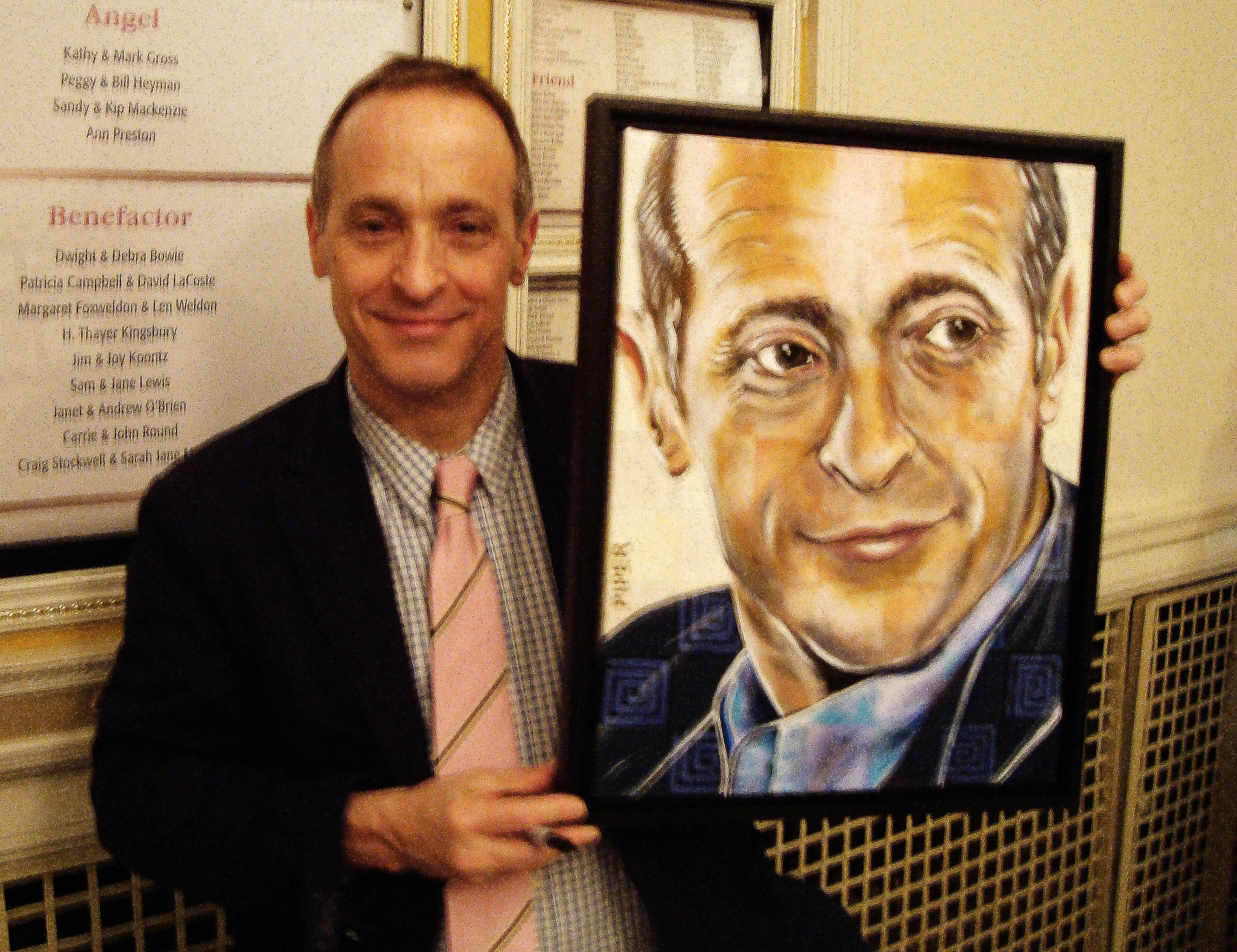In the image, we see David Sedaris standing on the left side, facing the camera and smiling. He is dressed in a black suit jacket over a white shirt adorned with blue lines forming a checkered pattern, and he wears a pink tie with thin yellow stripes. Sedaris has a receding hairline and dark eyes.

He is holding a framed self-portrait at the bottom with his right hand and on the side with his left hand. The portrait, encased in a black frame, shows him looking to the right, dressed in a blue jacket with a matching undershirt, capturing only his face and neck in a close-up view.

Behind Sedaris is a beige wall featuring framed papers. Two prominent framed items list names: one labeled "Angel," featuring Kathy and Mark Gross, Peggy and Bill Heyman, Sandy and Kip McKean, and Ann Preston; and the other labeled "Benefactor," listing Dwight and Deborah Bowie, and Patricia Campbell and David Laff. Other smaller, unreadable framed papers are also visible on the wall around him.